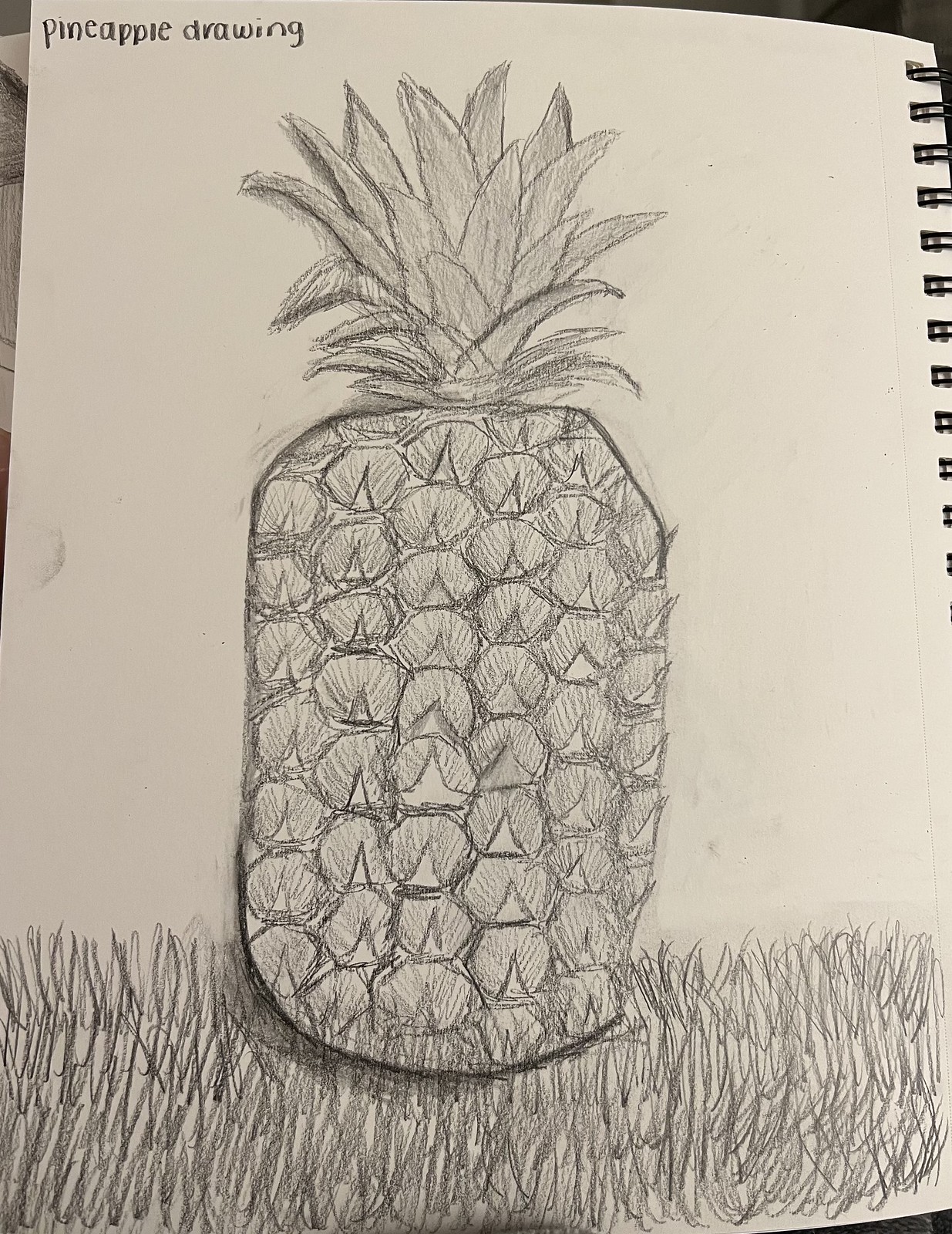In this detailed pencil sketch, we see a meticulously drawn pineapple resting on what appears to be a grassy area. The sketch resides in a spiral-bound sketchbook, as evidenced by the visible rings along the right edge of the paper. The top left-hand corner of the page bears the handwritten label "pineapple drawing." The illustration showcases an impressive level of detail, with substantial shading that enhances the contrast between the pineapple and the ground, giving it a realistic appearance. The pineapple features large tufts of leaves at the top, and the overall depiction is so precise and lifelike that it even evokes the iconic appearance of SpongeBob's house, albeit without the whimsical door and windows. The background remains plain and white, further focusing attention on the well-executed pencil work.